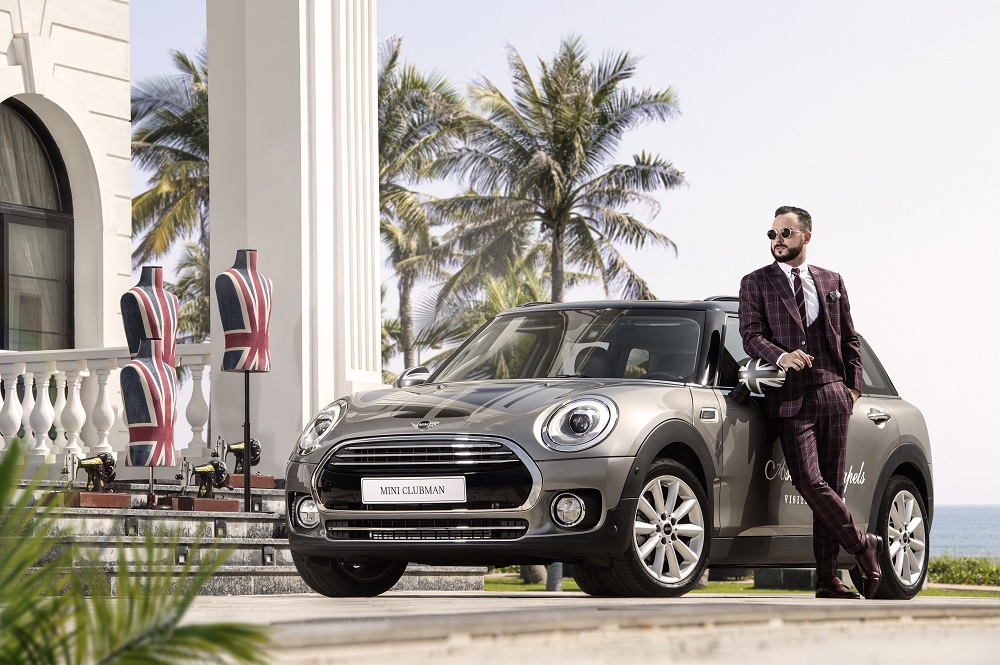In this striking photograph, a sharply dressed man in a red plaid suit and rounded sunglasses leans casually against a silver-grey Mini Cooper, reminiscent of the iconic car from "The Italian Job." He rests his arm on the side view mirror of the driver's side, gazing downward. Behind him, under a clear sky dotted with white clouds, palm trees sway gently, and the distant sea glimmers. To the right of the man, three headless mannequins draped with the Union Jack stand beside a grand white column, leading to a white building with a concrete block archway and a columned porch. A small plant adds a touch of greenery to the otherwise regal scene. The car, sleek and sporty with a Mini Clubman emblem on the front, is unoccupied, suggesting the man as its likely driver.